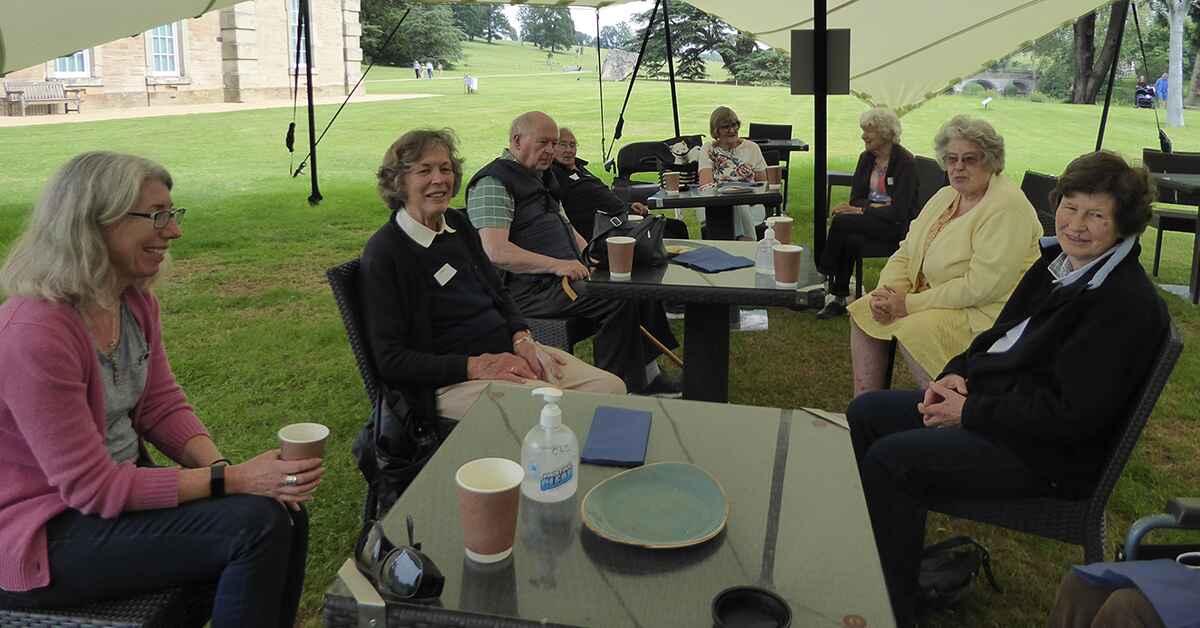The photograph captures a group of mostly elderly individuals, around their 70s and 80s, comfortably seated under a large canopy on a green lawn. There are eight people in the image, predominantly older women with one man among them. The setting appears to be a park-like area, featuring grassy hills, trees, and in the background, a structure with windows. The scene is well-lit yet flat, suggesting overcast weather. Multiple tables and chairs are arranged under the tent, and the individuals are seated around them, some looking directly at the camera while others engage with each other or focus on a speaker not shown in the frame.

Distinctive details include a prominent lady in a yellow dress with very white hair, adding a pop of color against the greenery. The image also shows various hues such as black, white, gray, brown, and shades of purple. On the table in the foreground, there's a large bottle of Purell hand sanitizer and several paper coffee cups, indicating a casual, relaxed atmosphere with people sipping coffee. Some individuals wear name tags, suggesting this might be an organized event, possibly a retreat or a social gathering. Despite the sizable canopy hinting at a larger anticipated attendance, the current scene appears intimate with only these eight attendees.